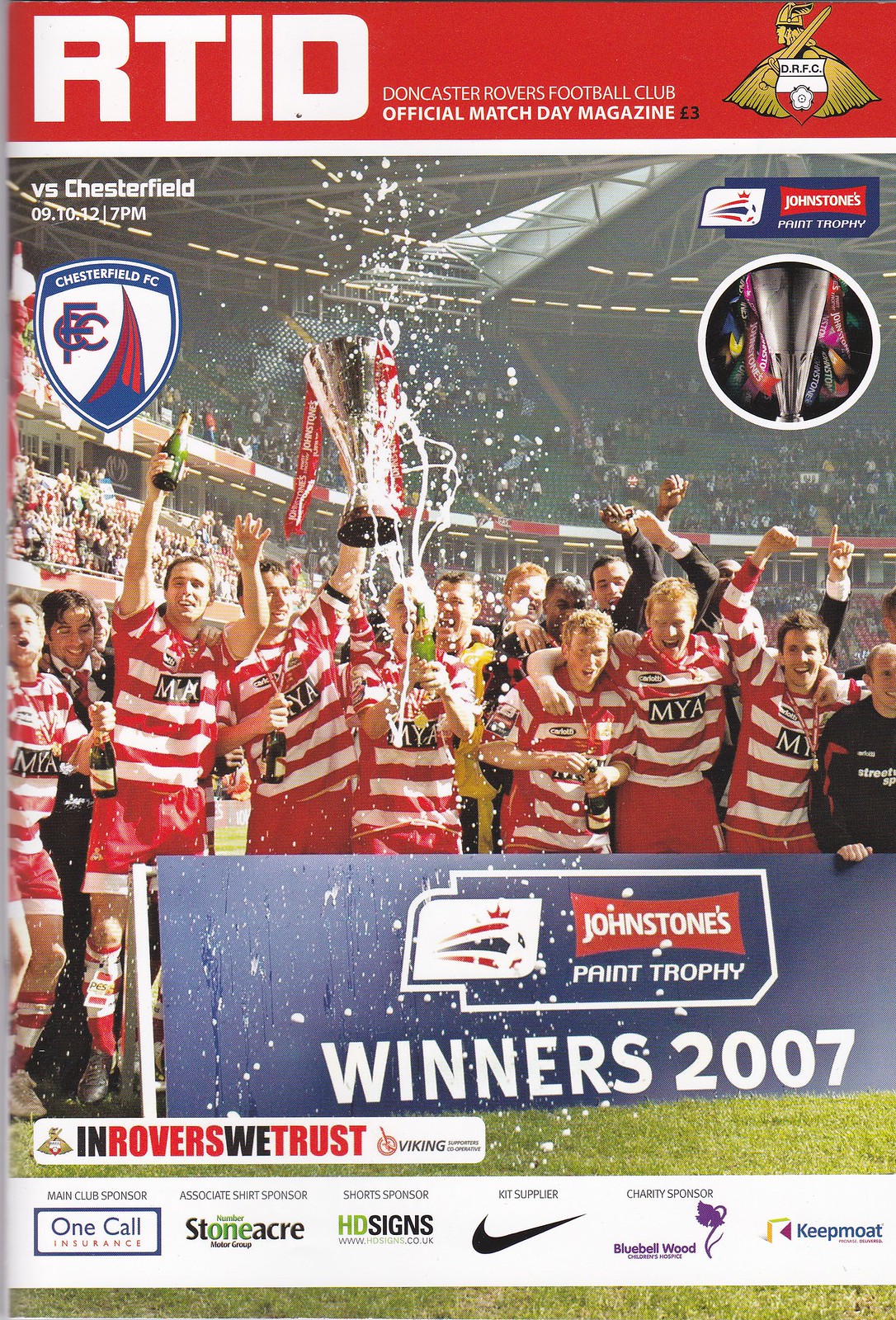The image is an advertisement for the Doncaster Rovers Football Club Official Match Day Magazine. At the top, it prominently displays "R.T.I.D." on a red background with white text, followed by "Doncaster Rovers Football Club Official Match Day Magazine." The price is indicated as three pounds or three euros. Next to this is an illustration of a Spartan warrior wearing a gold helmet with wings, holding a gold sword, and a red and white shield. Below this, there is a photograph of the Doncaster Rovers soccer team celebrating their victory in the 2007 Johnstone's Paint Trophy final against Chesterfield, as indicated by the text "versus Chesterfield 09 10 12 7 p.m." on the left side of the image. The team, dressed in red and white striped uniforms with "M.Y.A." logos on their shirts, is seen holding the trophy aloft amidst a cheering crowd and popping champagne. 

In front of them, there is a barricade with a sign reading "Johnstone's Paint Trophy Winners 2007." Further detailing includes a blue, white, and red badge for Chesterfield FC and another badge featuring a trophy symbolizing the Johnstone's Paint Trophy. Along the bottom of the image, the slogan "In Rovers We Trust" is inscribed. The lower section also features multiple logos, including the main club sponsor One Call Insurance, associate shirt sponsor Stoneacre, short sponsor HD Signs, kit supplier Nike, charity sponsor Bluebell Wood, and Keep Moat, as well as a purple flower-related sponsor. The background shows the audience stands filled with fans, highlighting the team's triumphant moment.